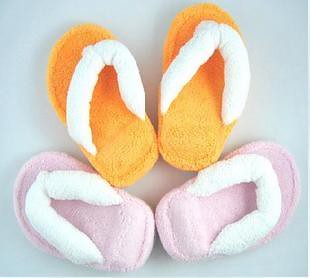This photograph features two pairs of fluffy, flip-flop style slippers situated against a pale blue-gray background. The slippers appear soft and plush, ideal for comfortable wear. The pair at the bottom are light pink with a white fluffy strap that crosses the foot. These slippers are arranged heel to heel, forming an exaggerated V shape. Above them lies the bright orange pair, which shares an identical design featuring a white strap. The orange slippers are positioned more conventionally, side by side, although one is perfectly straight while the other is angled slightly to the left. Both pairs are of the same size and contribute to a cozy, inviting image.